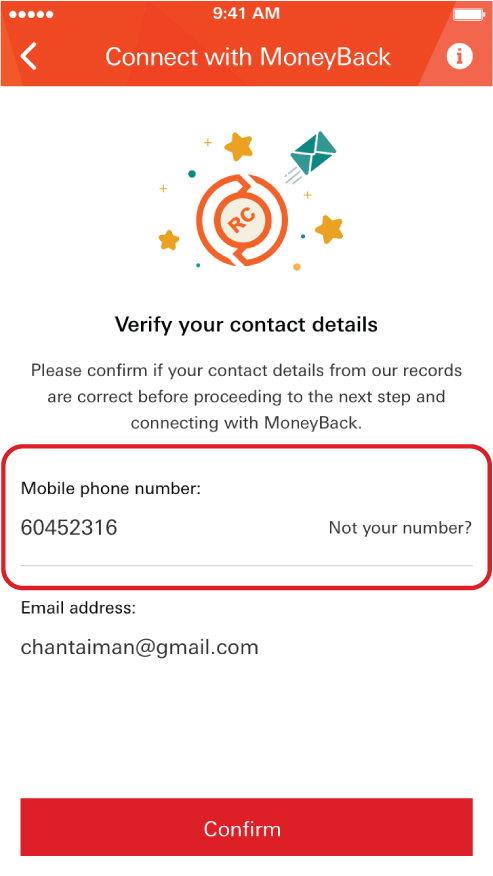This image shows a detailed view of a cell phone screen interface. 

At the very top, there is a reddish band where the status icons are displayed. On the left side, a set of three dots indicates the cell signal strength. In the center, "9:41 AM" is displayed, and to the right, a full battery icon is visible. 

Below this, an interface element features a left-facing arrow on the left, the text "Connect with Money Back" in the center, and an eye icon within a white circle on the right.

Further down, there is an emblem featuring "RC" in the middle of a circle, surrounded by three stars and an envelope icon rendered in green, which appears to be in motion. The background is adorned with various decorative elements, including green, yellow, and gold stars and circles. 

The main content area has a white background and displays a prompt: "Verify your contact details. Please confirm if your contact details from our records are correct before proceeding to the next step. Connecting with Money Back." 

Below this message, the mobile phone number “604-52316” is displayed, with a prompt to the right asking, “Not your number?” 

This section is within a red-bordered rectangle with rounded corners. Immediately below this rectangle, it says, "Email address, chantiaman@gmail.com."

At the bottom of the screen, there is a large red "Confirm" button.